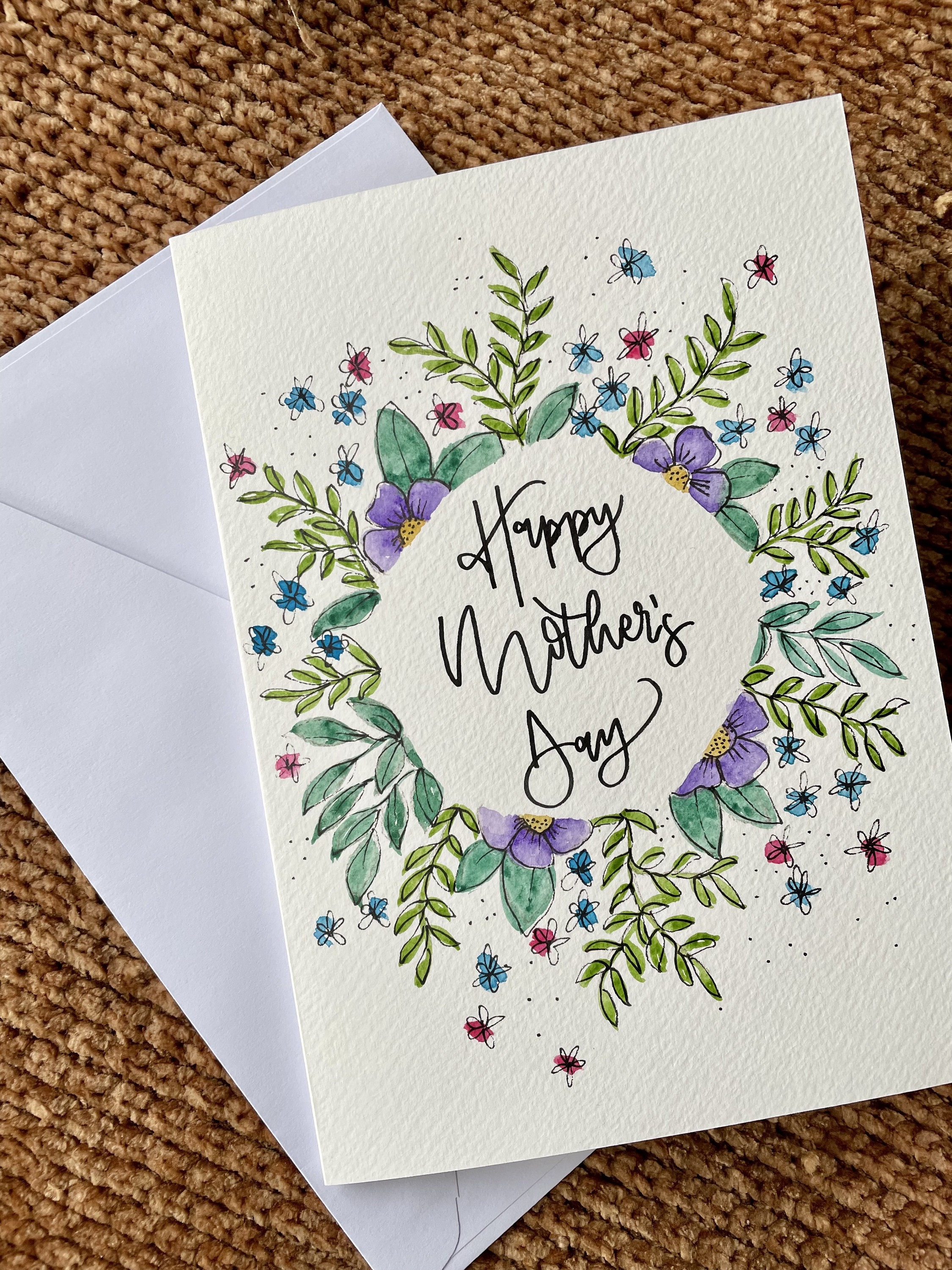This color photograph in portrait mode captures a charming Mother's Day card positioned atop a light brown and oatmeal-colored knit or crocheted material backdrop. The scene features a white envelope, placed diagonally beneath the card, with its back flap partially visible. The cream-colored card, designed to resemble textured white paper, showcases the words "Happy Mother's Day" elegantly written in black script at its center. Surrounding the script is a delightful ring of hand-drawn or watercolor-style flowers, predominantly purple with yellow centers, interspersed with green leaves and accentuated by subtle black outlines. Additionally, smaller flowers in red, light blue, and pink hues adorn the card, creating a vibrant and visually appealing bouquet. The card is slightly angled, enhancing its prominence as it occupies the center of the composition. The intricate and delicate floral artwork gives the card a heartfelt handmade aesthetic, making it a perfect centerpiece for celebrating Mother's Day.